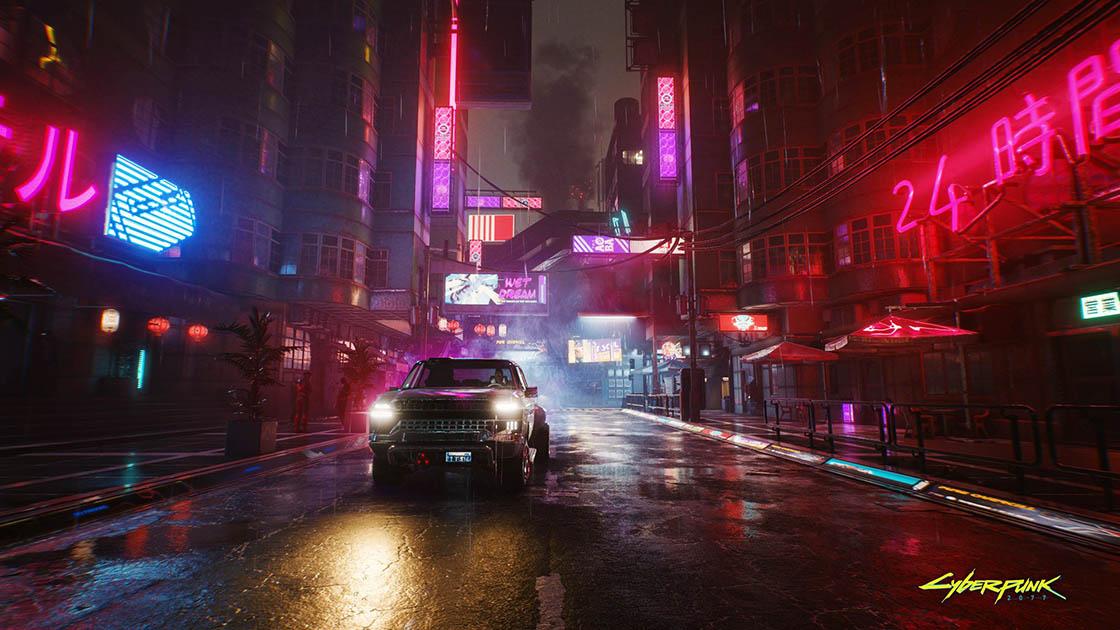This is a highly detailed photograph of a futuristic city street at night, brightly illuminated by numerous neon lights and signs. The wet pavement reflects the vibrant colors, suggesting it recently rained. Dominating the scene is a mix of pink, magenta, orange, and blue neon signs adorning buildings on both sides of the street. A dark car with its headlights on is approaching, casting a yellow glow onto the slick road. Notably, to the right, a prominent neon sign displays the number '24' accompanied by Asian characters, hinting at an East Asian setting. Above and around, more neon signs stretch across the street, some suspended between buildings. In the distance, tall, rounded apartment buildings with many windows are visible, shrouded in a subtle haze of smoke. Smaller details include red umbrellas on one side and Chinese lanterns hanging from a building on the other. At the bottom right corner of the image, the word "Cyberpunk" is visibly emblazoned in a striking yellow font.